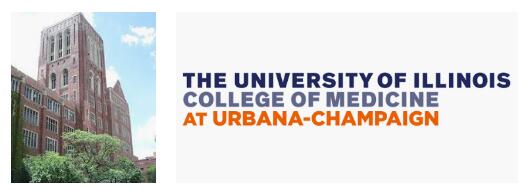This landscape-oriented screenshot, likely taken from a laptop, is divided into two distinct columns. The left column features a high-quality, professionally-taken photograph of the University of Illinois College of Medicine building at Urbana-Champaign. The building appears to be a tall, six-story structure, captured on a bright, sunny day, as indicated by the almost entirely white, bright upper left-hand corner and a blue sky with white clouds in the upper right-hand corner. A lush green tree spans the bottom left to bottom right, suggesting that the photo was taken in the summertime.

The right column, set against a gray rectangular background, features a series of text rows. The first row showcases the "University of Illinois" in dark blue text. Below it, the next row displays "College of Medicine" in gray, followed by "at Urbana-Champaign" in vibrant orange. This text column and the photograph are surrounded by a white background, creating a clear and clean visual separation between the two columns. The image is an informative visual representation used to advertise and promote the University of Illinois College of Medicine at Urbana-Champaign.